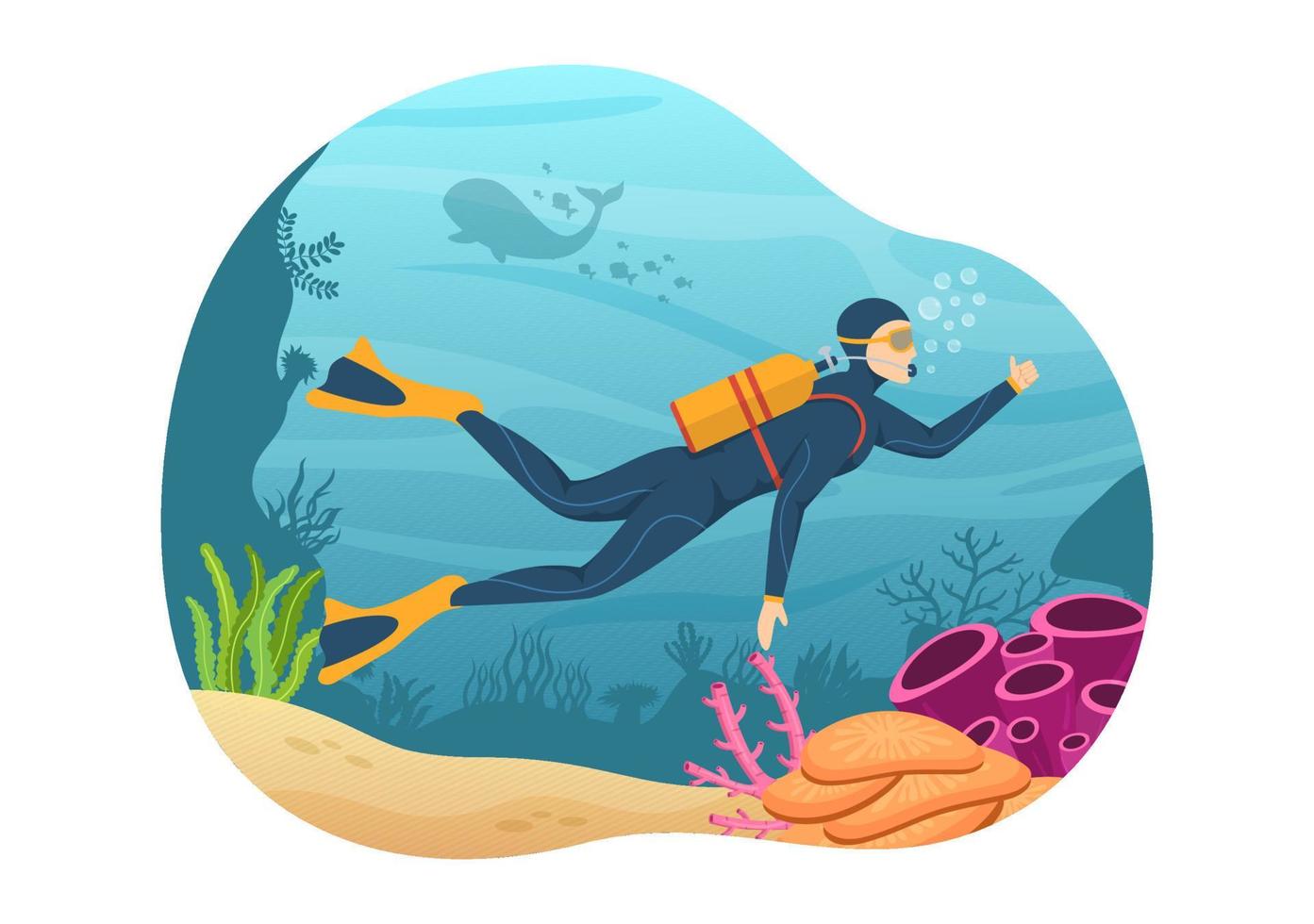This image is a computer-generated, cartoonish depiction of an underwater scene shaped like a droplet. The background, filled with various shades of blue, features the silhouettes of a whale accompanied by a school of fish. The seafloor below is covered with yellowish sand, with green seaweed in the bottom left corner and a variety of corals on the right. These corals include orange, pancake-like formations, light pink branches, and darker pink tube-like structures. 

In the foreground, a scuba diver, clad in a dark blue suit with yellow fins and a yellow tank striped with red, swims to the right. The diver, who is exhaling small bubbles, wears a mask and has their left hand raised in a thumbs-up gesture. Surrounding the diver are scattered blue rock formations, and the overall scene is filled with a playful, animated aesthetic.